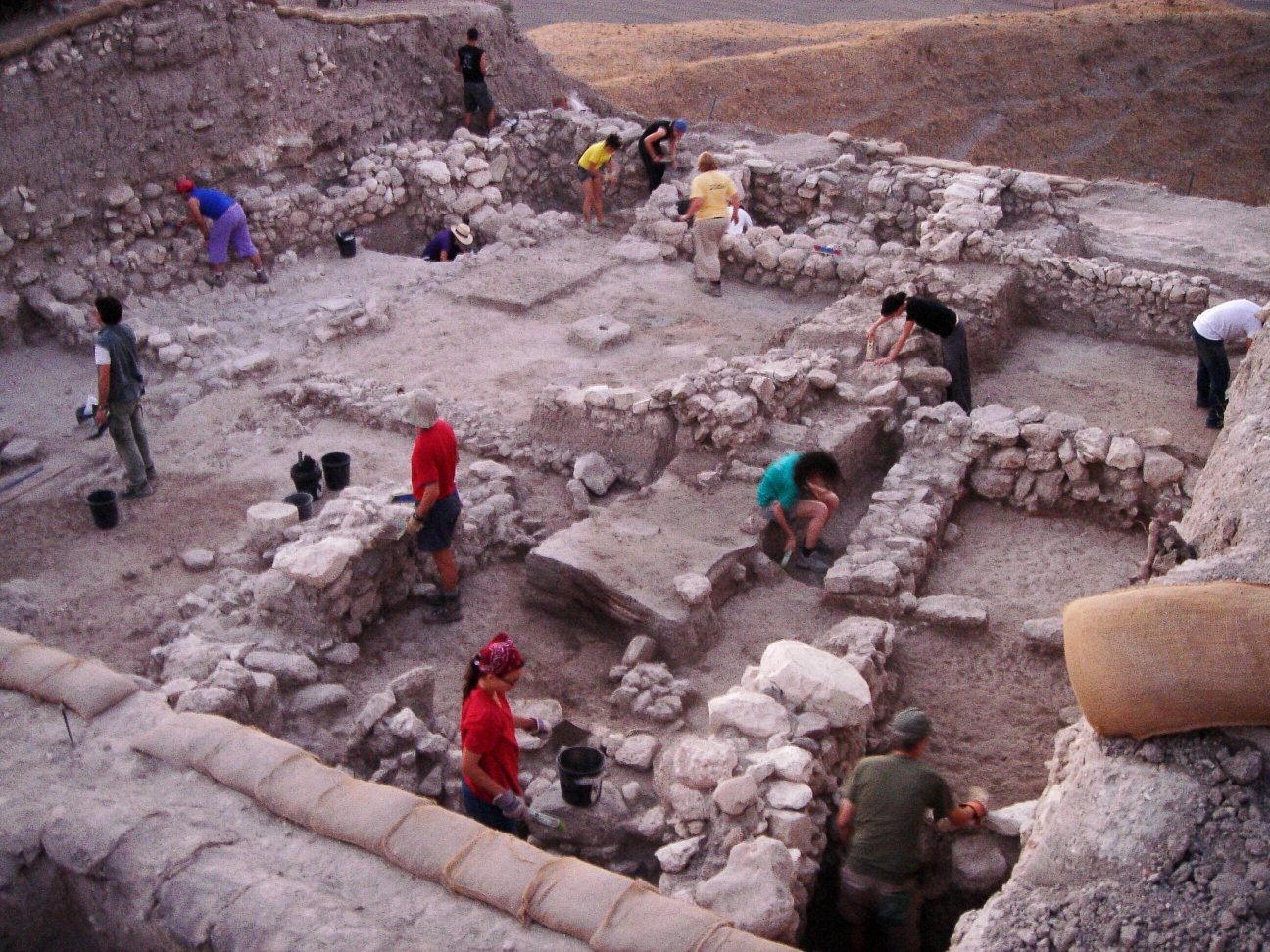This photograph captures an archaeologically rich excavation site teeming with activity. Around 11 to 13 archaeologists are meticulously working to unearth what appears to be ancient stone walls or dwellings. The site is a predominantly barren landscape characterized by tans, browns, and beiges, evoking a desert-like backdrop, especially visible in the top right corner where brown hills stretch out. 

The vibrant hues of the workers' attire punctuate the otherwise muted color scheme; bright reds, yellows, blues, and greens stand out against the earthy tones. Some workers don head and eye coverings as they engage in various tasks—some are actively digging, others sifting through the sand, and a few examining findings. A figure at the center is deep within an excavated section, hinting at the depth and complexity of the dig. Bags of sand are scattered in the foreground, indicative of the meticulous process of uncovering historical artifacts. Encircling the area, an outer stone wall forms a boundary, framing this hive of archaeological activity.